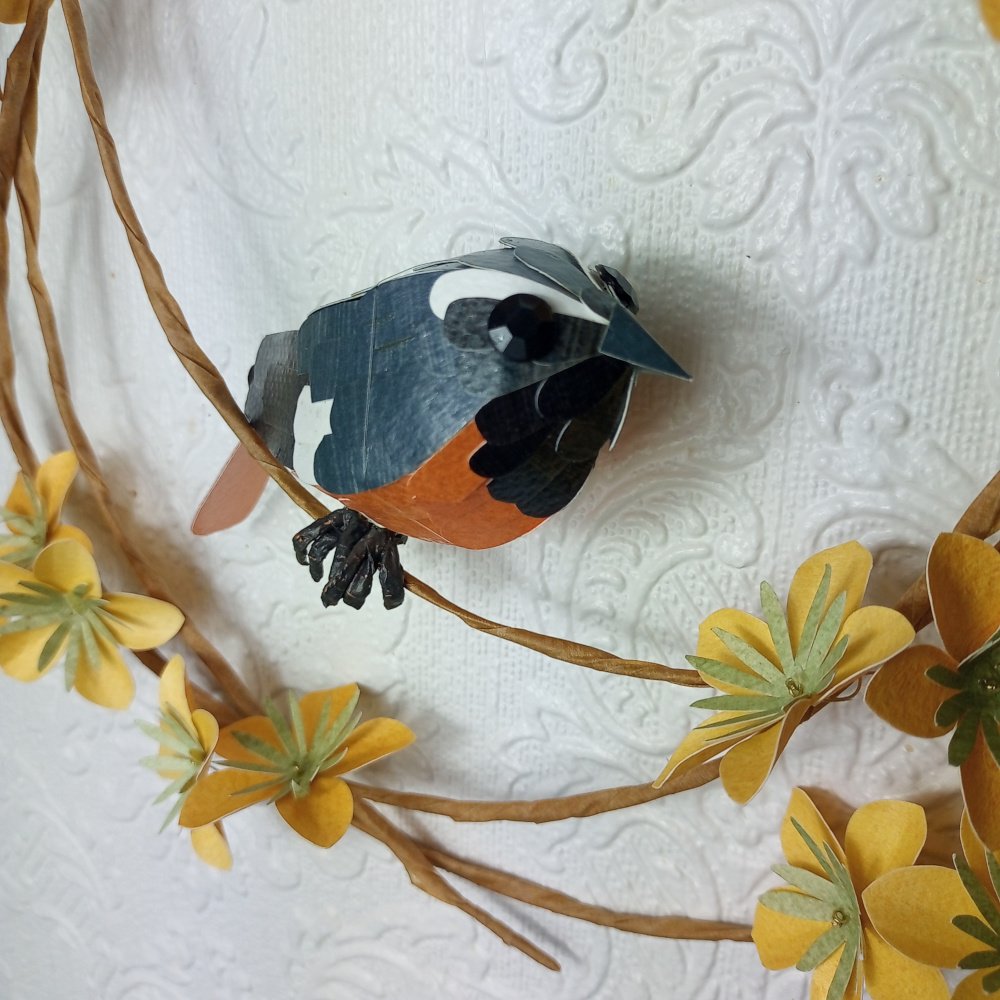This square photograph, measuring approximately six inches by six inches, captures an intricately crafted scene set against a textured white background adorned with beaded embroidery featuring leaf and spiral patterns. The foreground showcases a white dining mat with floral designs, upon which lies a handmade arrangement representing tree branches made from twisted and looped brown paper. These branches cascade from the upper left corner, downwards, and curl back upwards, predominantly occupying the right middle section of the image. Delicately perched on the topmost branch, a small bird made of paper or cardboard is posed, its head turned to the right and its boxy body detailed with individually crafted feathers. The bird is adorned with a black beak, black feathers on its chest, a red belly, light gray sides, black feet, and striking black bead eyes. Complementing the scene, the branches are decorated with at least five yellow flowers with green centers, made from paper, contributing to the whimsical and meticulous craftsmanship of the piece.